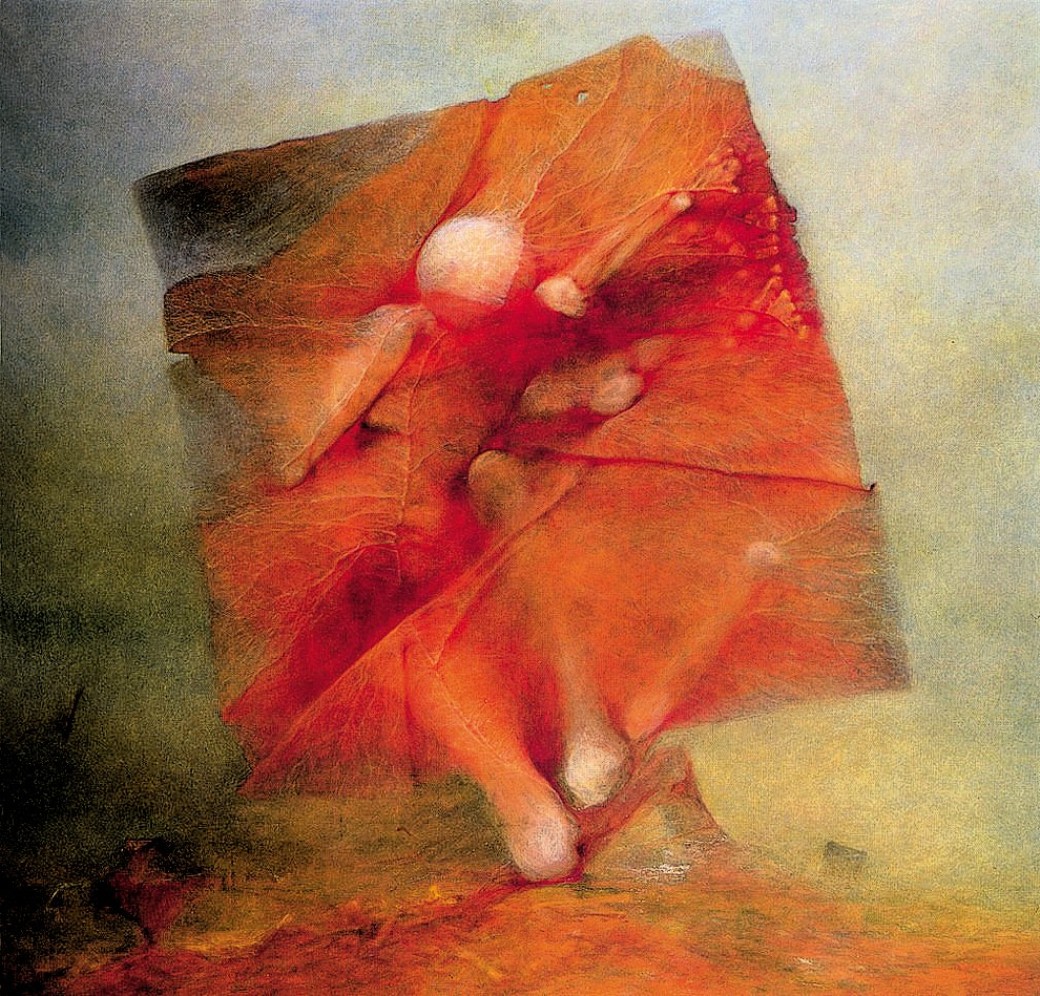The painting, with its modern and surreal aesthetic, features a complex interplay of colors and shapes. The background transitions from a pale light green and blue on the right to a darker green on the left. Central to the artwork is an off-centered, crinkled square in a peachy rosy color, reminiscent of tissue or crumpled paper. This square holds a translucent, layered figure that appears to have a rounded head, arms, and legs positioned within the square; the figure is rendered in varying shades of dark red and orange, creating a sense of depth and translucency. The left arm of the figure is raised towards the top of the square, adding to the dynamic composition. Surrounding the central square, the background morphs from gray at the top to darker shades at the bottom, while the right side shifts from yellowish black to a gradient of yellow, orange, and fiery red, evoking a vision of lava and fire. This compelling mixture of geometric and organic elements captures a striking, modern vibe open to various interpretations.